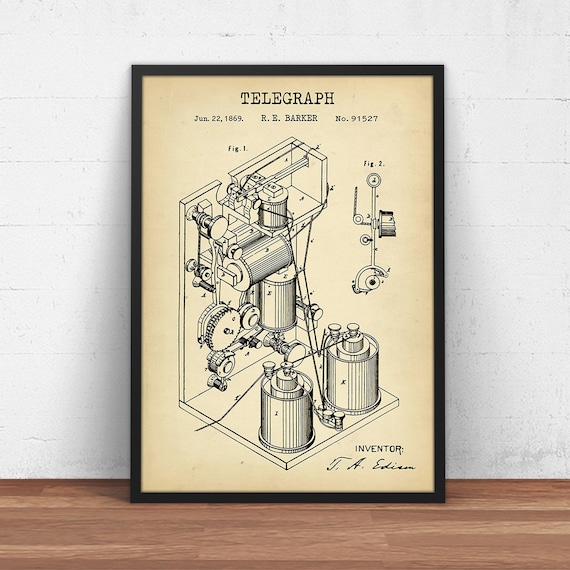The image is a detailed mock-up photo positioned against a white wall with painted wood planks and resting on a brown wooden floor. The mock-up itself is framed in a plain black frame, showcasing a vintage or reprinted diagram of a telegraph. The header at the top of the drawing labels it as "Telegraph," with the date of June 22, 1869, credited to R.E. Barker, number 91527. Central to the diagram, Figure 1 illustrates the various parts of the telegraph, including an L-shaped platform with multiple cylinders, gears, and wires, while Figure 2, located on the right side, focuses on the sender component of the mechanism. The lower right-hand corner of the drawing includes the word "Inventor" followed by a signature in script reading "T.A. Edison," indicating Thomas A. Edison's involvement in the creation or commissioning of this schematic.